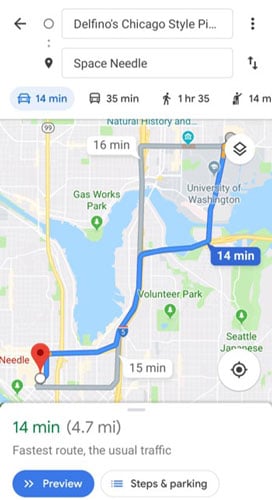**Detailed Screenshot Description:**

The screenshot is from Google Maps, with a minimalist interface design. At the top of the screen, the background is white, featuring a prominent back arrow pointing to the left. The arrow is black, sitting within a circular element that is white on the inside with a black border. Below the arrow circle, there are two gray dots, followed by another black spot with a white circle inside it.

Next to these elements are two vertically-stacked rectangles with white backgrounds and gray outlines. The first rectangle contains the text "Divino, Chicago style, PI..." in black, likely referring to "pizza." Below this, "Space Needle" is written. Adjacent to this text, three black dots (ellipsis) signify additional options.

Continuing downward, there are two arrows: one pointing up and the other down, both in black. These are probably navigation options or directions indicators.

The next row features transportation information, starting with a blue "O4" and an icon of a darker blue car next to it, indicating some form of travel mode. The figure "14 min" may refer to a duration. To the right, there's an icon of a bus or train paired with "35 min." Following this, a black walking stick figure indicates it takes "1H35" or one hour and thirty-five minutes on foot. Additionally, an icon showing a raised hand suggests a taxi option with the number "14," although the information cuts off here.

Below these elements, the main map portion is visible, predominantly featuring blue areas representing water bodies and green areas for parks and natural spaces. Key locations such as "Seattle Japanese Garden," "Volunteer Park," and "Gas Works Park" are marked in green. The streets are depicted in gray with white lines. A blue navigation line traces a route from the starting point to the Space Needle, with an annotation in green reading "14 minutes (4.7 miles) via usual traffic."

Overall, the screenshot efficiently combines navigational tools with visual geographic information, highlighting major landmarks and estimated time to the destination in vibrant colors against a clean design.